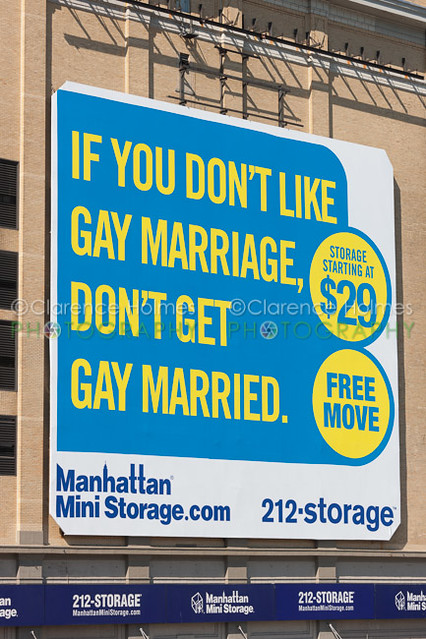The image is a large advertisement mounted on the side of an older, sand-colored brick or stone building with decorative faux columns. The ad features a prominent social message and commercial information. The white sign, with each corner cut off, takes up about half the height of the tall, rectangular building. The top section of the sign has a turquoise blue text box with yellow sans-serif text that reads, "If you don't like gay marriage, don't get gay married," making a humorous and progressive statement. Below this message, there is a yellow circle with a blue border stating "Storage starting at $29," and another yellow circle with a blue border advertising a "Free move." At the bottom left of the sign, the website "manhattanministorage.com" and the phone number "212-STORAGE" are displayed. The sign is high on the building, with the awning for the actual Manhattan Mini Storage service visible below, although the ground floor is out of the frame.